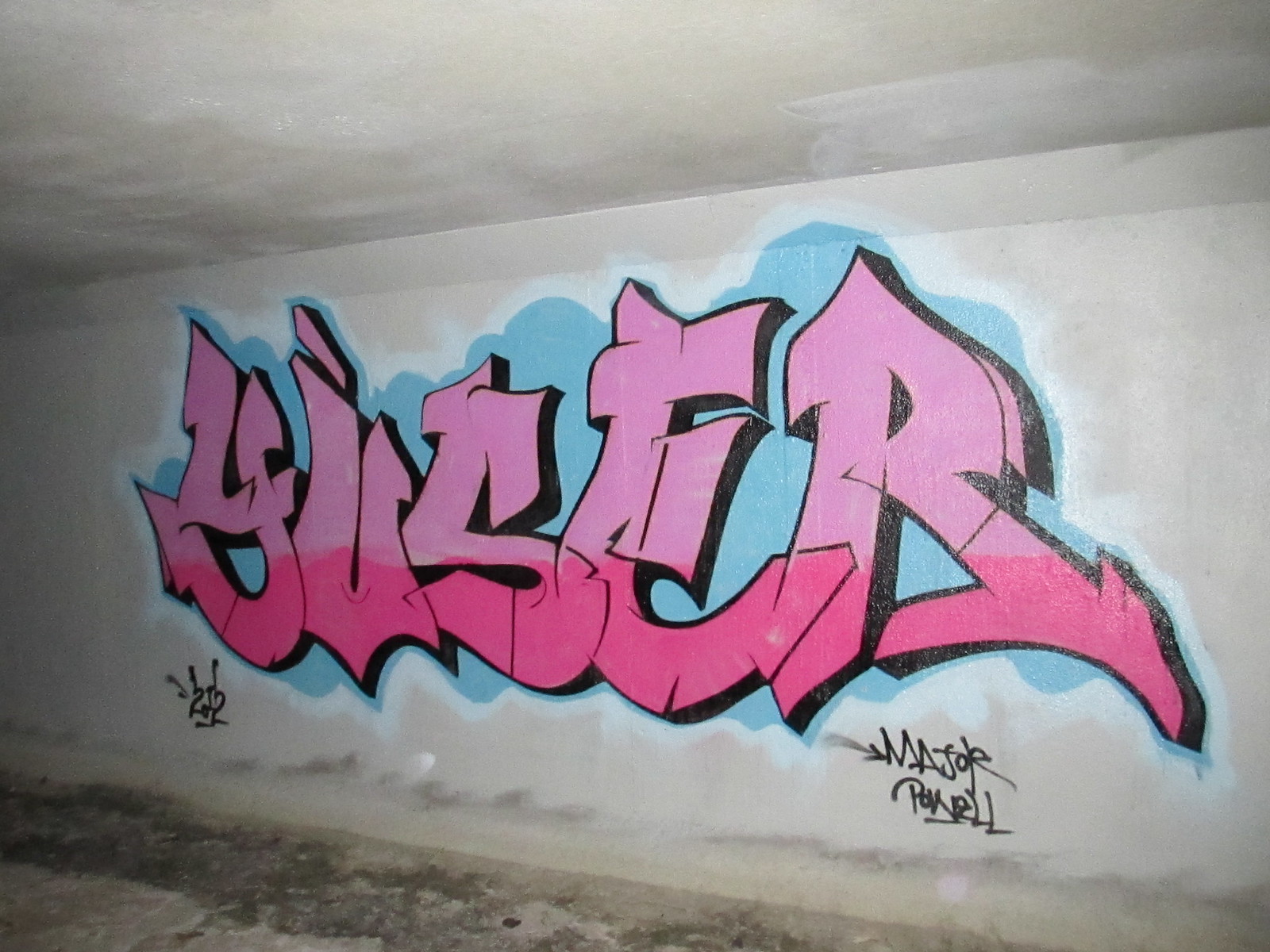The image captures a scene which could be indoors or the exterior of a tunnel, featuring a graffiti painted on a gray concrete wall. Above, a white ceiling is visible, indicating that the location might be covered. The ground appears worn and weathered, suggesting an exposed environment.

Dominating the wall is an intricate piece of graffiti with the text "BUSTER" or perhaps "ABUSER," characterized by thick, vibrant letters. The upper half of each letter is painted in a light pink, while the lower half is in a darker pink, outlined boldly in black. A cloudy blue background encircles and diffuses behind the letters, giving a floating effect.

In the bottom right-hand corner of the graffiti, the words "Major Pakel" are tagged in black spray paint. Additionally, to the left of the graffiti, there is another graphic that reads "2 and a Half." The scene also depicts potential water stains or mold at the bottom of the wall, indicating age or ongoing exposure to the elements. 

Overall, the photograph combines elements of decay and urban artistry, with details like the freshly painted or spackled ceiling adding layers of contrast and depth to the setting.